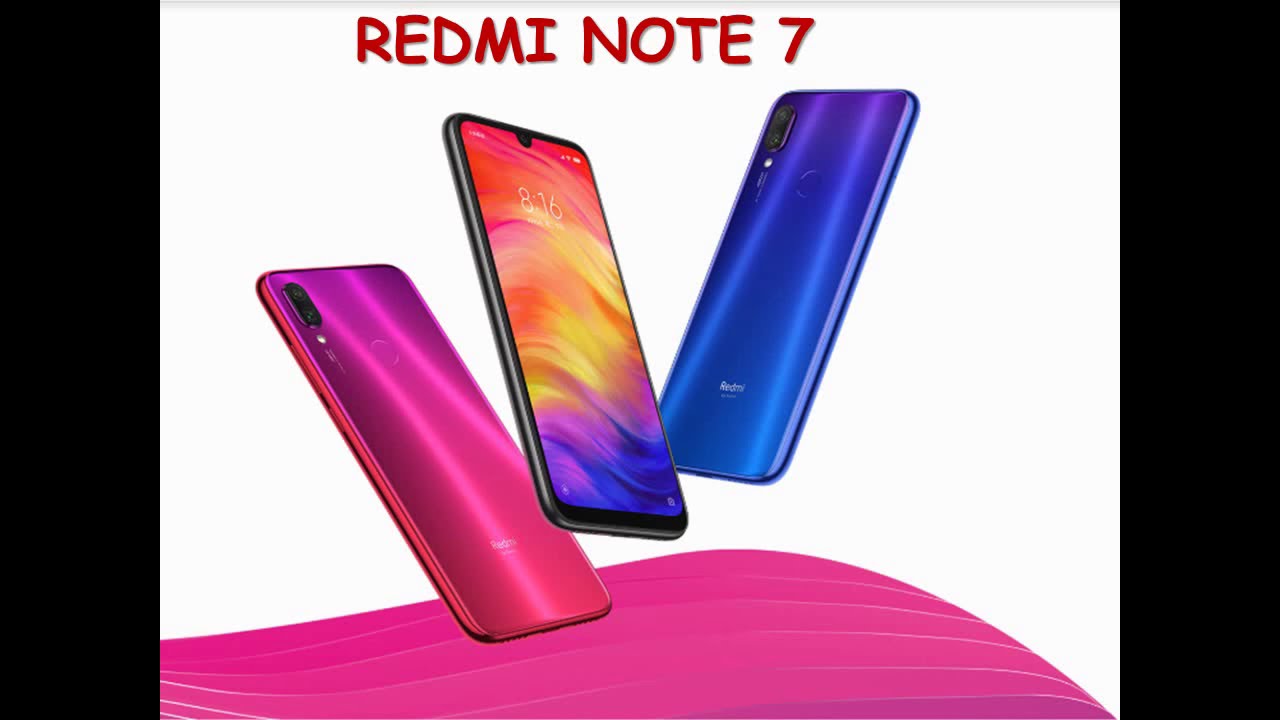The image is a graphical advertisement for the smartphone model "REDMI NOTE 7," with the model name displayed across the top in uppercase, red text against a white background. Below this text, three smartphones appear to be floating. The phone on the far left showcases its back, displaying a gradient from pink at the bottom to purple at the top with some glowing pink lines. The phone in the center presents its screen, which features colorful waves—purple at the bottom, transitioning to yellow and then red near the top—and displays the time "8:16" in white text. The phone on the right reveals its back, which is a glossy blue with streaks of purple. The bottom of the image features a swirly pink design, while black rectangles occupy the left and right edges, adding contrast to the composition.